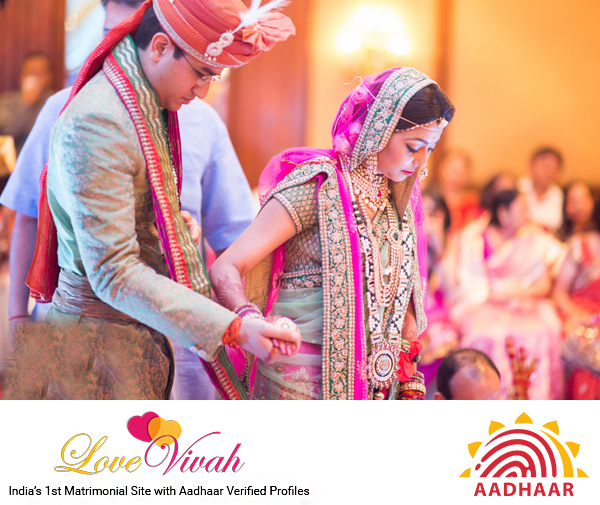This vibrant image appears to be from an Indian wedding or similar event. Central to the picture is a couple, with the man standing behind the woman, holding her hand and assisting her down some steps. The man is adorned in traditional Indian attire, featuring a high red turban-like hat with a white feather, a multicolored scarf, and garments in varying shades of green and red. The woman, likely the bride, wears a rich, pink hood and a pink and multicolored robe embellished with intricate beads and decorative elements. Her ensemble includes a gold headdress, numerous bracelets, and possible tattoos, adding to the vibrant tapestry of hues including pinks, greens, and blues. The background is softly blurred but reveals seated guests clad in traditional dresses, attentively watching the couple. A banner at the bottom-left corner of the image reads "Love Viva" in pink, adjacent to a yellow text declaring "India’s first matrimonial site with Aadhaar verified profiles," accompanied by a red and yellow heart.